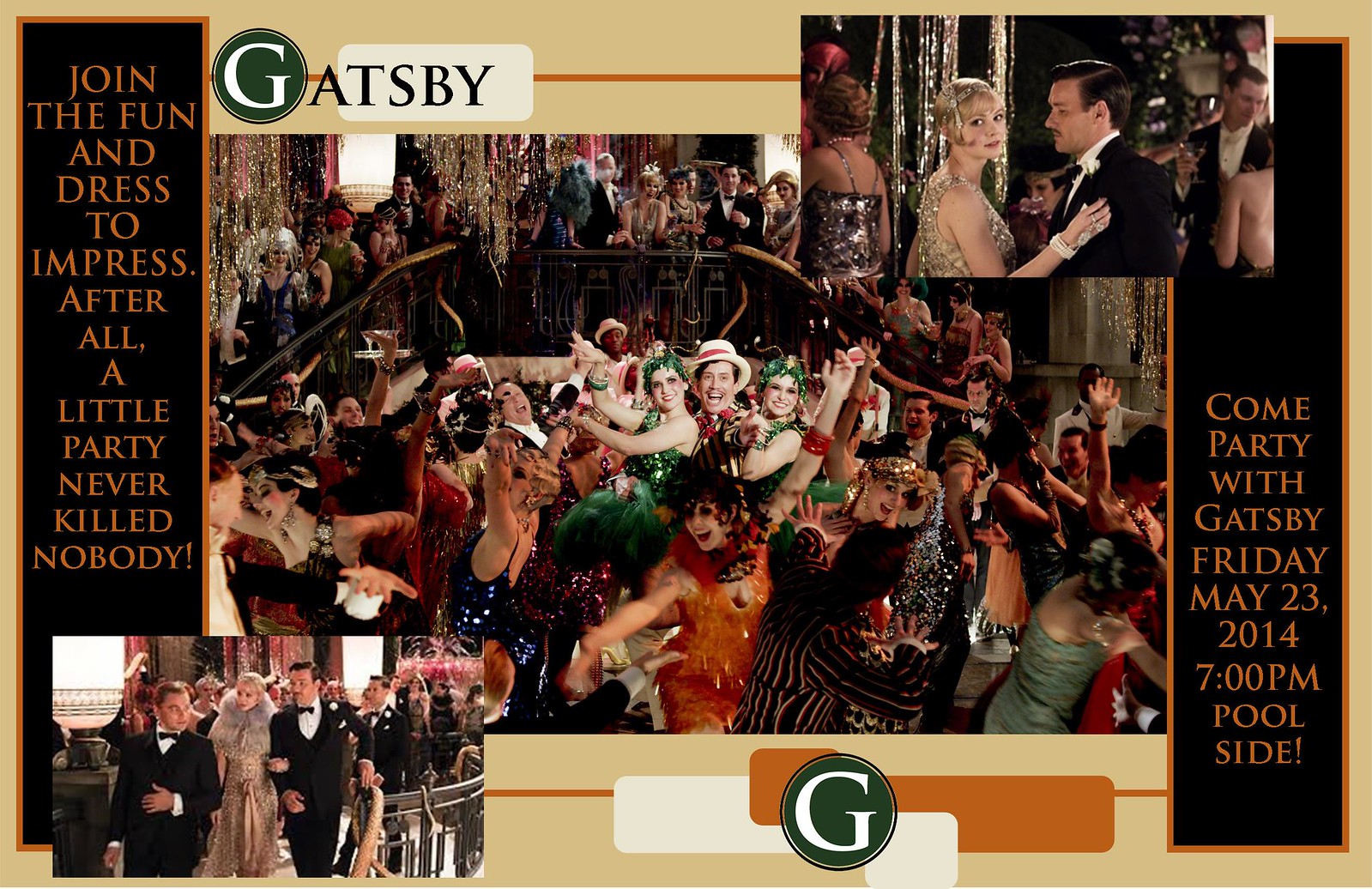This elegant poster serves as an exclusive invitation to a Great Gatsby-themed party, dated for Friday, May 23, 2014, at 7 p.m., to be held poolside. The background is predominantly beige with striking black rectangles framing the sides. The top of the poster prominently features the word "Gatsby," with a white 'G' encircled in green, positioned to the left. The tagline in the left rectangle reads in orange text: "Join the fun and dress to impress. After all, a little party never killed nobody." The right rectangle invites guests with, "Come party with Gatsby, Friday, May 23rd, 2014, 7 p.m., Poolside." The same white 'G' in a green circle reappears at the bottom center, overlaid on a pattern of orange and white rectangles. Central to the invitation are three vivid photographs of elegantly dressed individuals in 1920s or 1930s attire. These images, showcasing people dancing and celebrating in a formal, opulent setting, some on a grand staircase and others under a spotlight, vividly capture the essence of the glamorous Gatsby era. The dancers' vibrant dresses in blue, orange, green, and red stand out brilliantly. The overall design, with its black, gold, and yellow text on a sophisticated beige background, exudes vintage class and allure, perfectly setting the tone for an unforgettable evening.